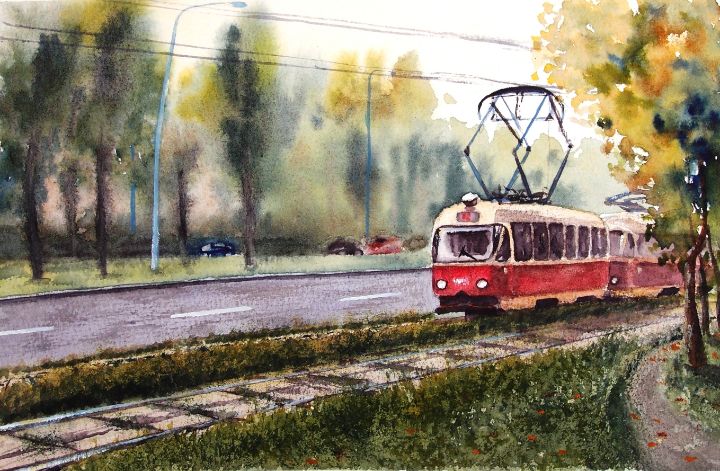This watercolor painting showcases a vivid scene of a red and cream-colored trolley gliding along a rail track that runs parallel to a street. The trolley features six windows on each side and a large windshield, with overhead cables that assist its movement. Below the trolley, the track is bordered by a grassy field scattered with fallen leaves, hinting at the changing seasons from summer to fall.

To the left of the trolley, a streetlight stands beside a marked road, while off in the distance, blurry, dark, and light green trees stretch from the horizon. The sky above is a pale white, subtly contrasting with the autumnal hues of the scene. The background is a mix of muddled and splotchy trees, adding depth and a sense of distance, while parked cars are faintly visible in the distance, evoking a serene suburban setting. The overall composition is enhanced by the artist's skillful use of colors, blending oranges, blues, and varying shades of green to create a picturesque and tranquil atmosphere.